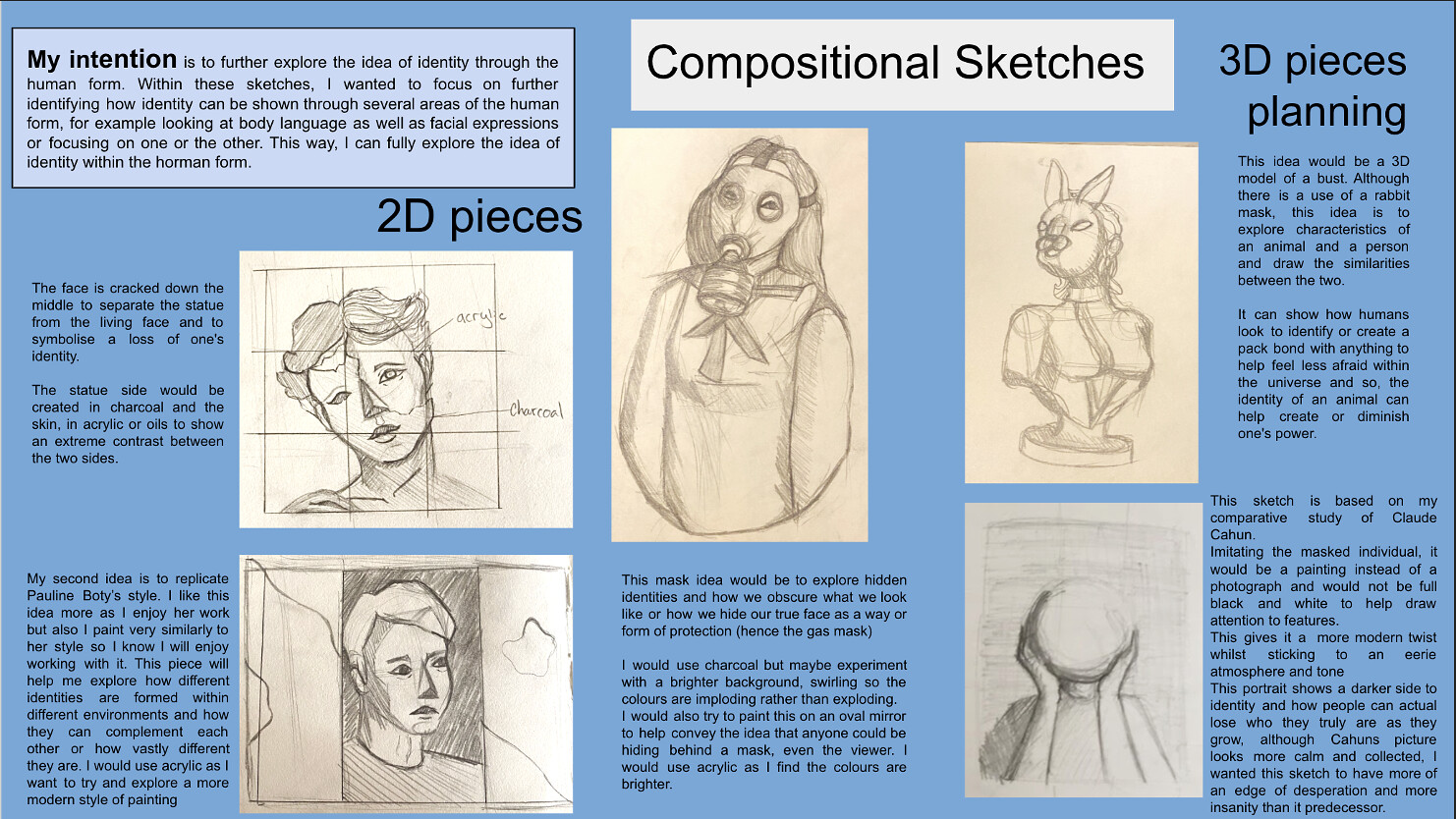The image displays a landscape-oriented page from an instructional leaflet titled "Compositional Sketches" highlighted in a central white rectangle with black text set against a blue background. The page is framed with a pinstripe black border running horizontally along the top and vertically down the right side. In the upper left corner, a light blue rectangle with a black outline contains a statement of intention, reading: "My intention is to further explore the idea of identity through the human form. Within these sketches, I wanted to focus on further identifying how identity can be shown through several areas of the human form. For example, looking at body language as well as the facial expressions of focusing on one or the other. This way I can fully explore the idea of identity within the human form." 

The page is divided into sections: "2D Pieces," featuring sketches with accompanying descriptive text explaining the techniques and ideas. One sketch shows a face within a grid pattern, while another depicts a head sectioned like a window pane. Below the main title are three distinct sketches: a woman in a gas mask, a bust of a person wearing rabbit ears, and another figure holding an empty circular space where the head should be. On the far right, under the label "3D Pieces, Planning," are more explanations and possibly additional sketches, though the text is too small to read clearly. Overall, the leaflet showcases a variety of sketch examples, including hand-drawn faces and surreal images, all intended to explore and communicate themes of identity through artistic expression.